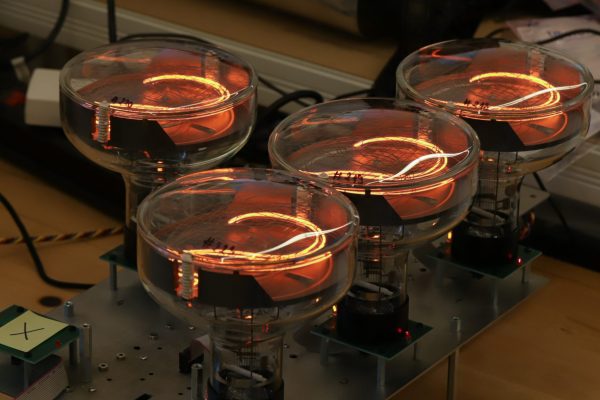The image showcases a close-up of intricate electrical equipment centered around four cylindrical, glass-encased coils, each mounted on a brown base and connected to a metal framework. These objects, which resemble truncated light bulbs, feature glowing filaments inside—illuminated in an orangish-red hue—and are surrounded by an array of cords and additional components. The setup appears to be situated on what may be the edge of a white or gray table. Notably, one of the devices at the bottom left has a green sticky note with a black X on it, adding a distinctive mark amidst the high-tech assembly.